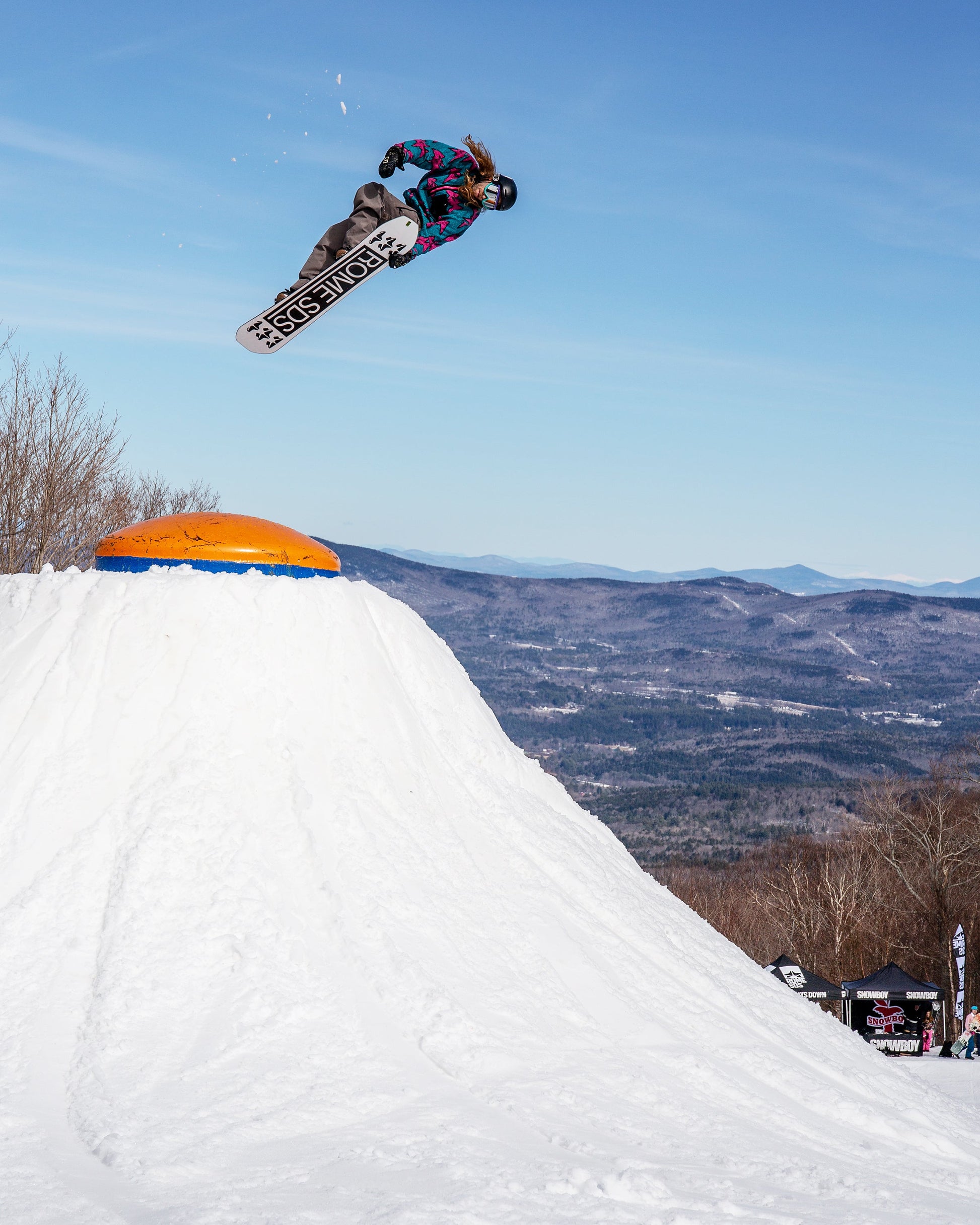In this dynamic photograph, a snowboarder clad in a red and blue anorak and a helmet is captured soaring above a snowy hill. The snowboarder, positioned slightly to the right of the image center, sports a white snowboard emblazoned with the black and white text "Rome SDS." The snow-covered hill, occupying the bottom left third of the image, leads the viewer's eye towards the expansive background where a range of blue-hued mountains stretches across the horizon. Below the hill, leafless trees dot the landscape, while to the right, a small blue structure crowned with an orange dome and a modest concession stand can be seen. The pristine blue sky above completes this exhilarating winter sports scene.